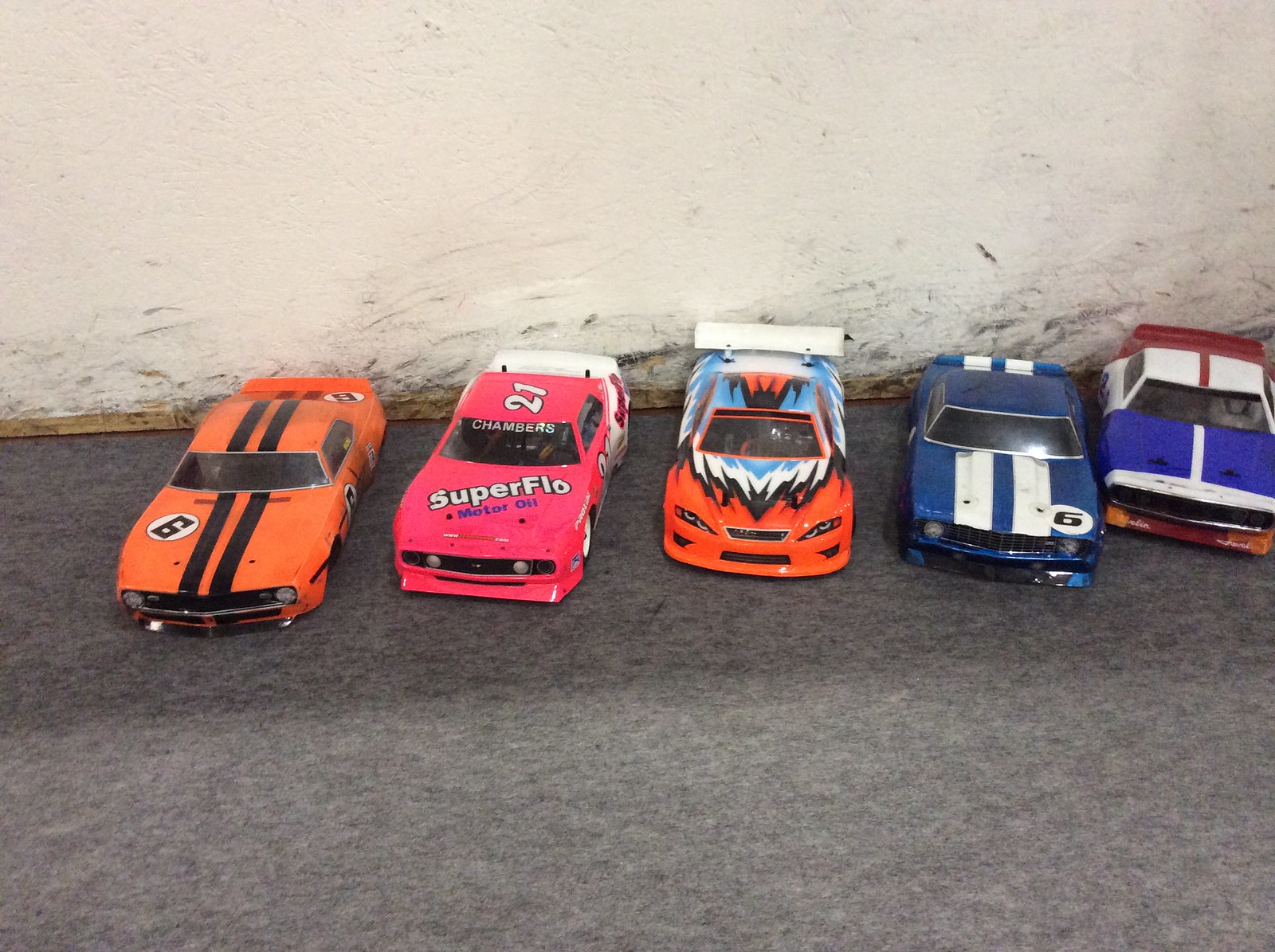This image captures five die-cast model cars aligned against a scuffed, white concrete wall on a gray mottled floor. Each car, appearing as scaled-down racing vehicles with a mix of metal and plastic bodies, vividly showcases unique designs and details:

1. On the far left, a striking orange car with dual black stripes extending from hood to boot, resembling a Dodge Charger or Challenger. This car prominently features the number 6.

2. Next, a pink car adorned with the text "Super Flow" and the number 21 on the hood. This vehicle also bears a white spoiler, enhancing its sporty look.

3. Positioned in the center, a multicolored car with a dynamic flame-like design in red, blue, black, and white hues. It has a white spoiler and stands out with its intricate detailing.

4. The fourth vehicle is a blue car with white racing stripes from the hood to the boot, likely another American model, possibly a Dodge, and also features the number 6.

5. Finally, partially captured on the far right, a white car with dual black panels on the hood, a red stripe along the roof, and a red spoiler. The car’s hood shows blue blocks with white stripes.

All cars are poised facing outward, exuding a sense of readiness against the stark backdrop, reminiscent of miniature NASCAR racers prepared for a track showdown.